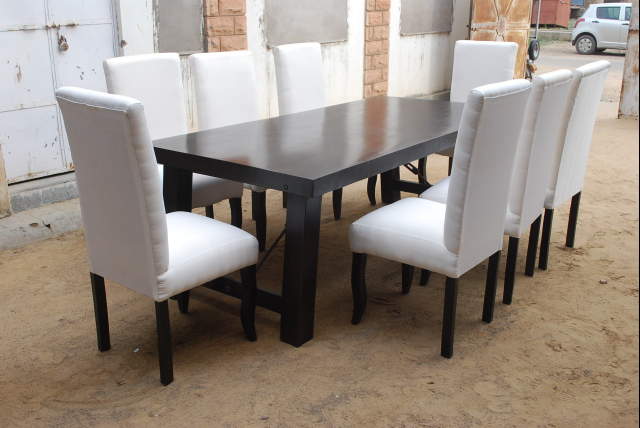The image depicts a large, rectangular, dark wooden dining table set outdoors on a dirt ground. The table features thick legs and is accompanied by eight high-back, white cushioned chairs, each sharing the same material and tone as the table. Three chairs are positioned along each length of the table, with one chair at each end. In the background, there is an old building made of tan brick with white accents, characterized by visible scuff marks and an entrance door. A white car and a small tire can also be seen in the background, suggesting a setting that might be a backyard or similar outdoor area.